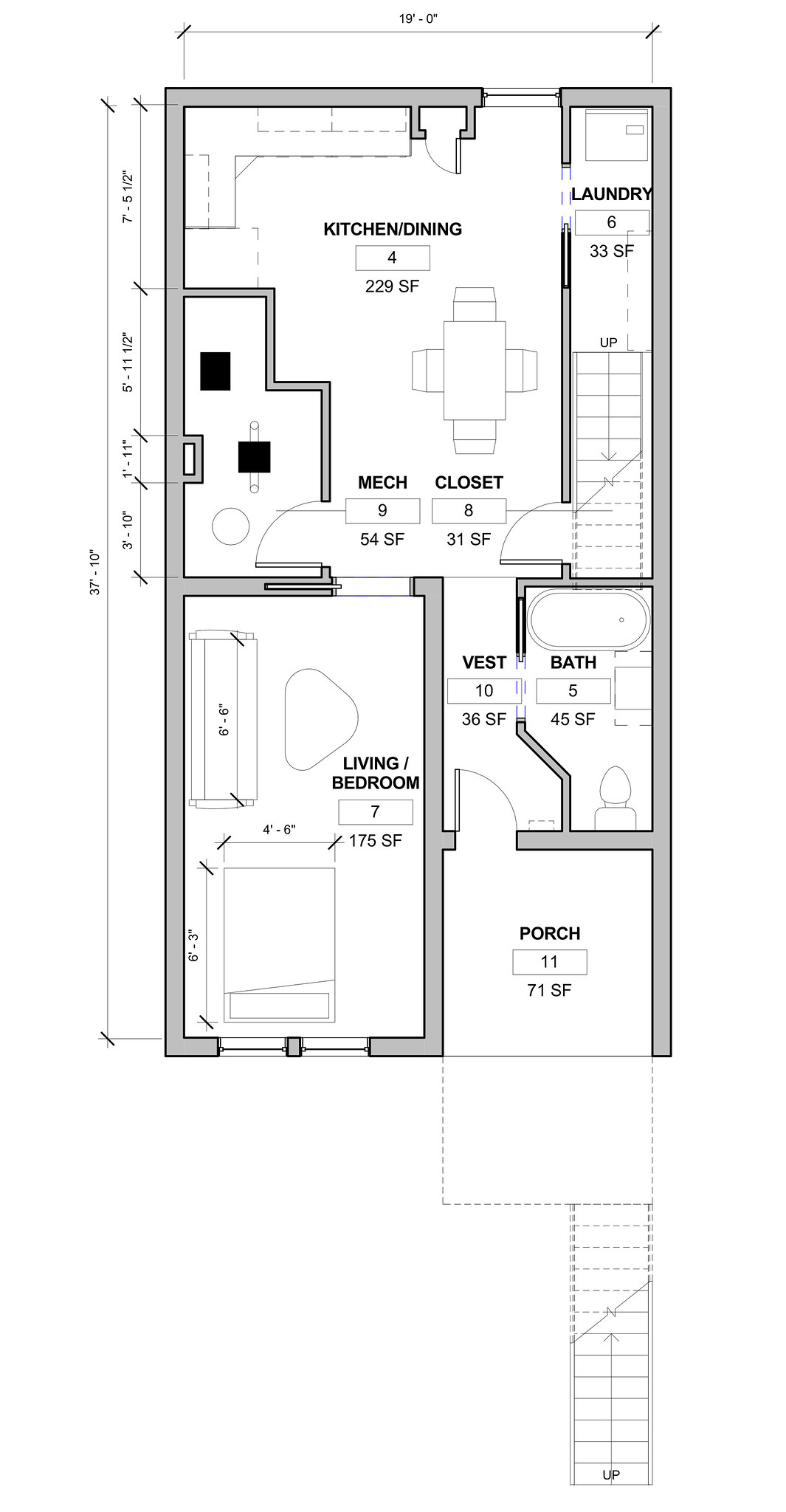Here is the cleaned-up and detailed caption for the image:

"The image shows a detailed blueprint of a house set against a white background. The blueprint includes various sections of the house annotated with measurements and labels. At the top section of the blueprint, measurements are indicated by lines, providing dimensions for parts of the structure. Similar measurements are also noted along the sides of the blueprint.

In the bottom right corner, the blueprint depicts a series of steps leading to a porch, which then transitions into an area labeled 'Vest.' To the right of this area is a room labeled 'Bath,' complete with illustrations of a bathtub, sink, and toilet. Adjacent to the bathroom is a 'MECH Closet,' indicating a mechanical closet.

Heading further up the blueprint, there is a room with a table, and next to it on the right is a section labeled 'Laundry.' The upper left corner of the blueprint indicates the presence of another room, though specific details are more challenging to discern.

Below this, there is yet another room. In the bottom left corner of the blueprint is the 'Living Room,' complete with representations of a couch and another unspecified object. The precise details of the furnishings and room layouts offer comprehensive insight into the design and functionality of the house."